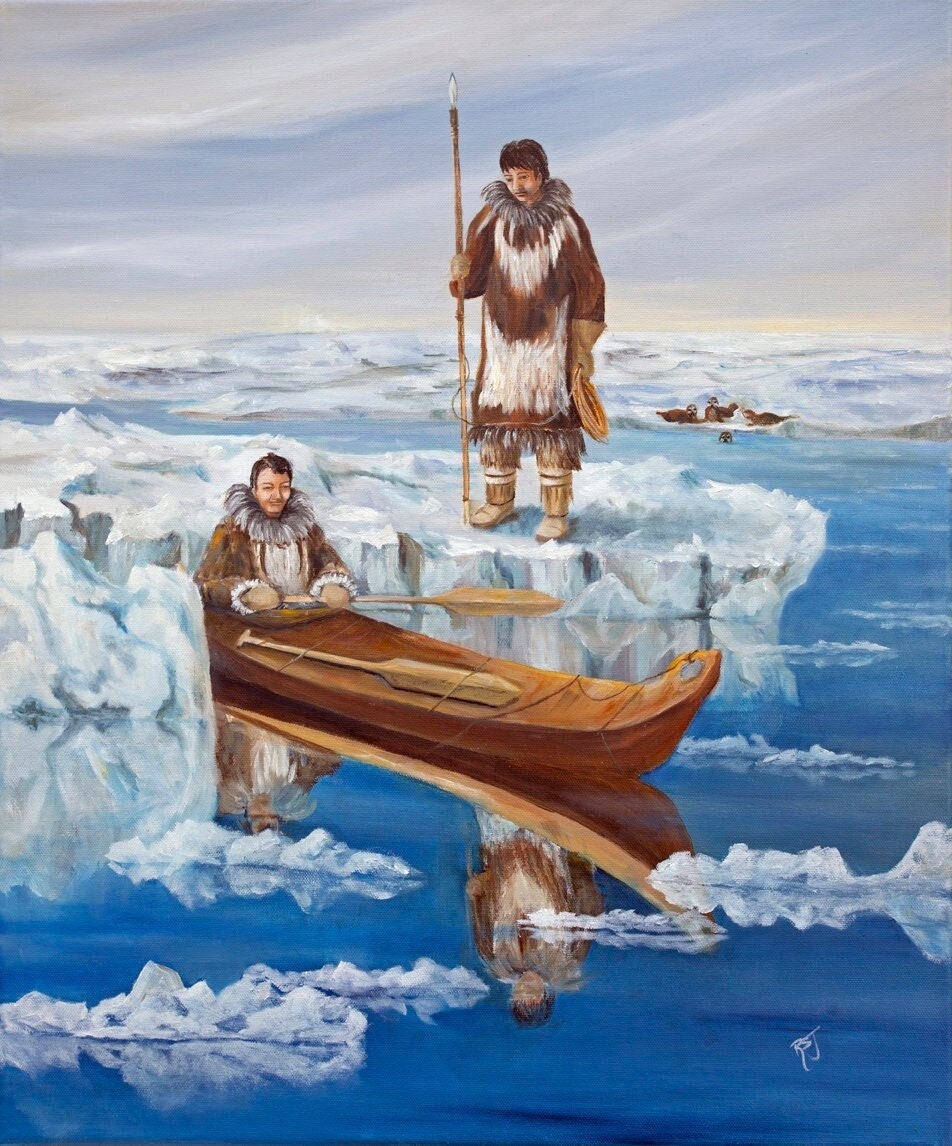This painting depicts a historical scene of two Eskimos dressed in traditional fur clothing. The setting is a cold, ice-laden environment with reflective blue water and patches of ice. In the foreground, one Eskimo is seated in a canoe, emerging from between blocks of ice, dressed in a brown fur coat with a gray fur ruffle around the neckline and brown mittens. His coat has white fur cuffs, and his reflection is visible in the still water below. Standing to his right is another Eskimo on a small iceberg or floating sheet of ice. He is clad in a brown and white fur jacket with a fluffy gray collar and tan boots, holding a tall spear with rope, likely for use as a harpoon. The sky above is a mix of hazy gray clouds and blue, adding to the serene yet cold atmosphere. In the background, four brown seals are depicted, three on the ice and one in the water, enhancing the painting's rich detail of native Alaskan life.